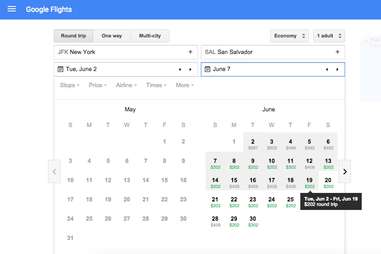The webpage seen in the image is designed primarily for Google Flights. At the top, there is a blue rectangle in the far left corner featuring three white horizontal lines. Next to it, the text "Google Flights" is displayed prominently. Below this header, there is a smaller section with black text that is not legible from the image provided.

Below this header, there are three horizontal rectangles across the page. The first of these rectangles on the far left includes text indicating flight options such as “Round-Trip,” “One-Way,” and “Multi-City.” Evidently, the option highlighted at this moment is “One-Way.”

Just beneath these tabs, there is a rectangular section with text displaying "New York" followed by "Tuesday, June 2nd." Further below, the page is divided into two calendar months—May on the left and June on the right. On the June calendar, the date range from June 2nd to June 19th is highlighted in light gray, suggesting a selection. The remaining dates are white, indicating they are not selected. 

A black tab appears under the date of June 19th, with small white text on it that is difficult to read. Below this, there is a note mentioning “June 2nd - round trip,” written in white text, but again, the specific contents are hardly legible due to the small font size.